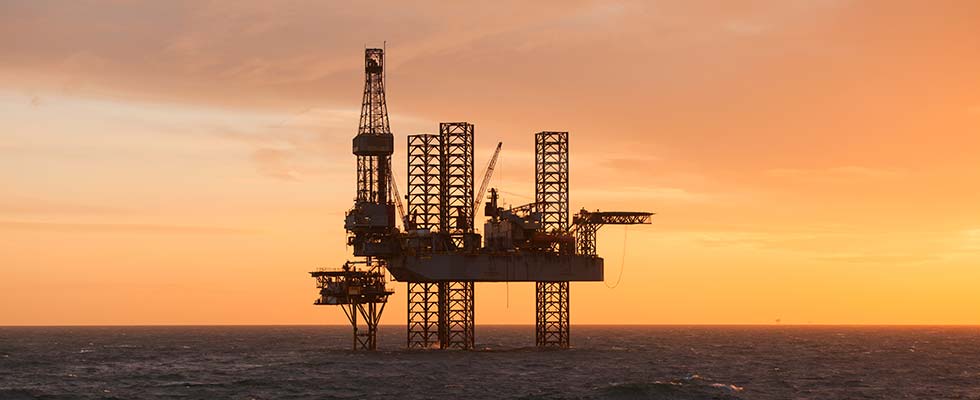This horizontally aligned rectangular photograph captures a vast expanse of the ocean at either dawn or dusk, evidenced by the stunning yellow-orange hues at the horizon blending into a grayish coral sky. The water below is relatively calm with a few choppy waves exhibiting white tips. Dominating the center of the image is an oil rig with multiple vertical metal columns supporting a large platform. The rig features several smaller concrete bases extending upward, with at least one crane angled towards the right. The sky occupies the upper two-thirds of the picture, showcasing a beautiful gradient from coral to deep orange and yellow near the horizon, while the ocean fills the bottom third with its brownish tinge and frothy waves. The entire scene is devoid of people, highlighting the isolation and majesty of the industrial structure amid the serene yet powerful seascape.